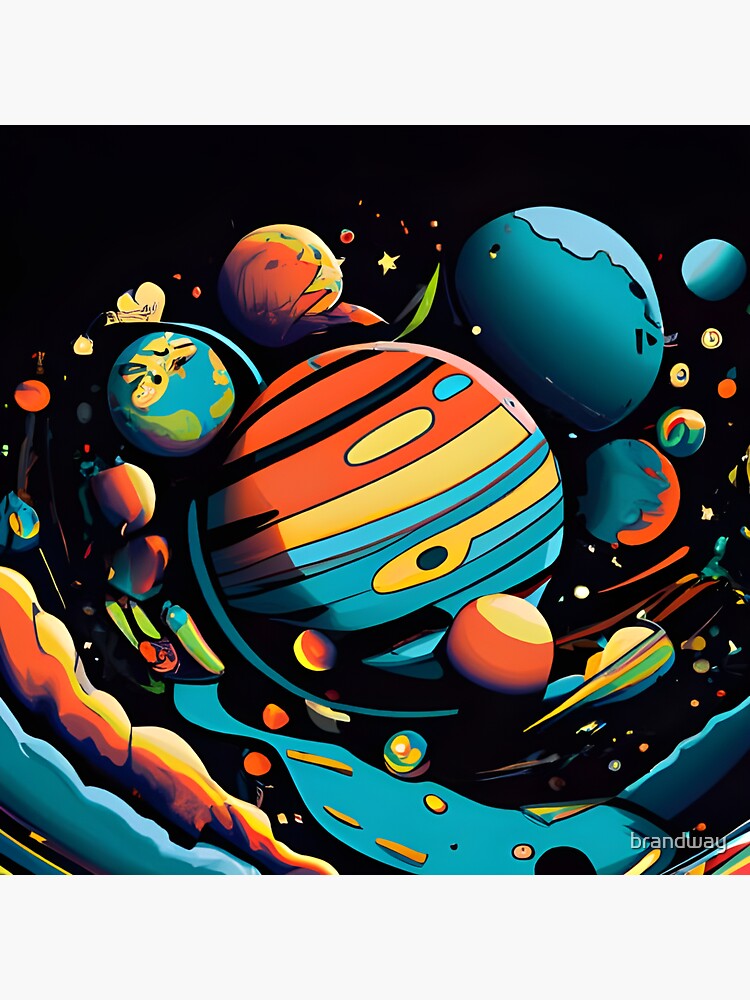This is a vibrant, abstract, cartoony space image with a plain black background, showcasing a cosmic scene filled with colorful spheres representing planets. At the center of the image is the largest planet, adorned with bands of red, yellow, and aqua stripes, surrounded by various other vibrant planets. Notable among them is an Earth-like planet with green continents and a blue ocean, as well as a predominantly green and light blue planet.

The planets, both large and small, appear to be swirling together amidst tiny spheres and stars that dot the background, adding a sense of movement to the scene. On the bottom left of the image, there is a segment resembling an amoeba-like shape floating in space and teal-colored clouds. In the foreground, an intricate yellow heart shape with fine black designs exists among small colorful planets, creating a swirling effect with multicolored debris.

At the bottom right corner of the image, the watermark "Brand Way" is visible in light blue lowercase letters, likely in a standard or Times New Roman font, suggesting a possible comic magazine origin.